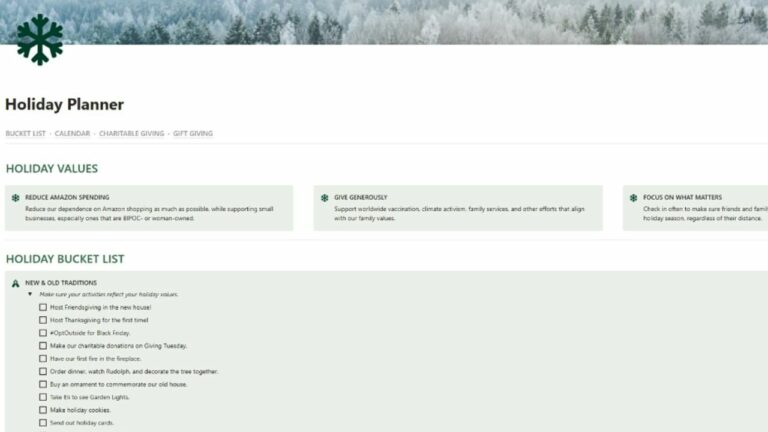The image is a screenshot of a planner website interface, prominently titled "Holiday Planner" at the top left corner. The interface is organized into several sections, each serving a distinct aspect of holiday planning. The sections labeled "Bucket List," "Calendar," "Charitable Giving," and "Gift Giving" are clearly visible. Within the "Holiday Values" section, there are key principles outlined: "Reduce Amazon Spending," "Give Generously," and "Focus on What Matters." Although specific descriptions under these principles are not easily readable, their presence is noted. Additionally, the "Holiday Bucket List" section features a heading "New and Old Traditions," accompanied by multiple fields with empty checkboxes to the left, indicating items or activities intended to be tracked or completed. The overall layout suggests a comprehensive tool for organizing and managing holiday-related activities and objectives.